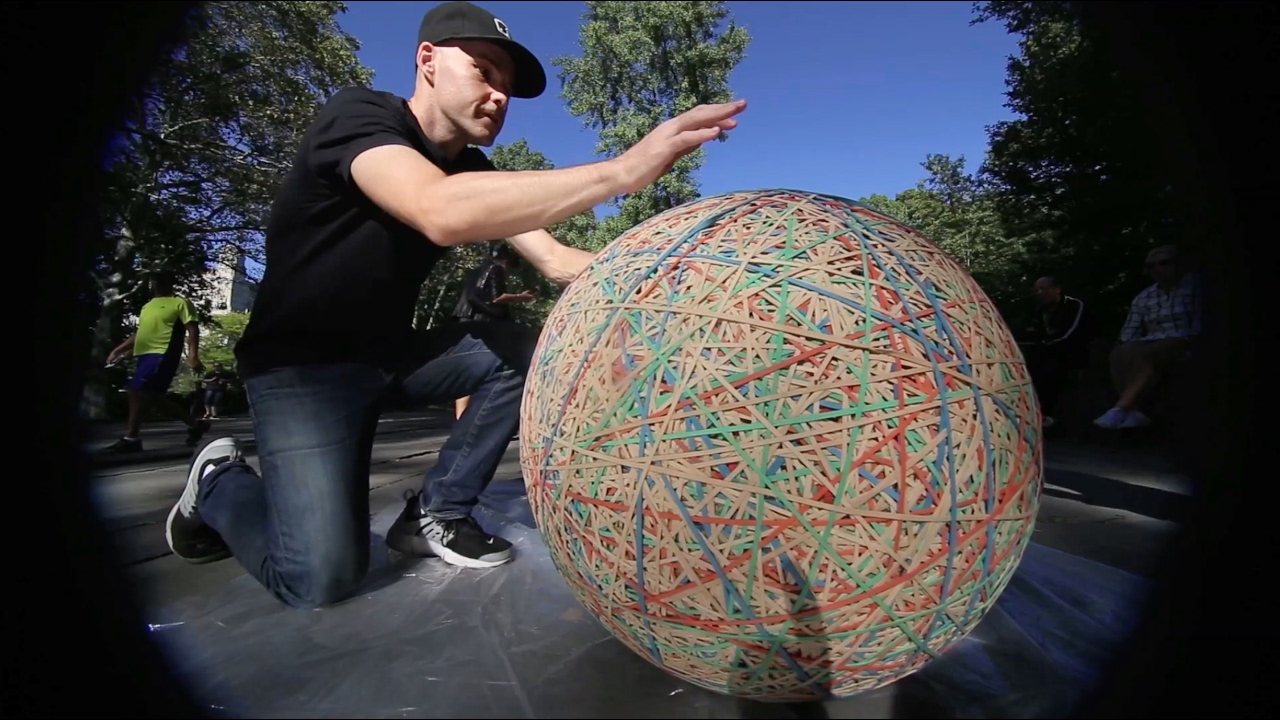This realistic photograph, shot with a fisheye lens or wide-angle perspective, features a distinctive vignette effect, where the edges fade into darkness, creating a circular focal point in the center. Set outdoors on a sunlit day with a clear blue sky and lush green trees in the background, the scene captures a man kneeling on a paved surface. The man, dressed in a black baseball cap, black t-shirt, dark jeans, and black and white athletic shoes, is interacting with an enormous rubber band ball, approximately one to three feet in diameter. The colorful ball, composed of traditional tan rubber bands interwoven with various shades of green, red, and blue, dominates the center of the image. The man is positioned on the left side of the ball, with his right knee on the ground and his left leg bent, his right arm resting on the ball while his left hand hovers above it, suggesting action or engagement with the object. The photograph has no text and might depict a world record attempt or an artistic interaction with the giant rubber band ball.